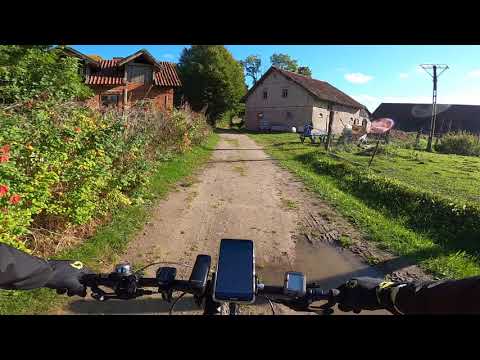This image captures a dirt driveway, flanked by grass, vegetation, weeds, and a notable mud puddle on its right side. The pathway seems to lead towards two distinct farmhouses—a brown brick house with old-style architecture on the left, and a seemingly dilapidated white stone house on the right. There might be a barn in the background as well. The shot is taken from a cyclist’s perspective, possibly from a helmet cam, as we can see the handlebars of an off-road bicycle adorned with various attachments including a smartphone, a GPS, and maybe an odometer or light. The cyclist is dressed in black gloves and a long-sleeved black shirt, maneuvering to avoid the mud puddle. Ahead, the scene is framed by a blue sky sprinkled with a few clouds, a solitary tree, and a telephone pole in the distance. The overall atmosphere suggests a quiet, rural setting that may be either in use or potentially abandoned.